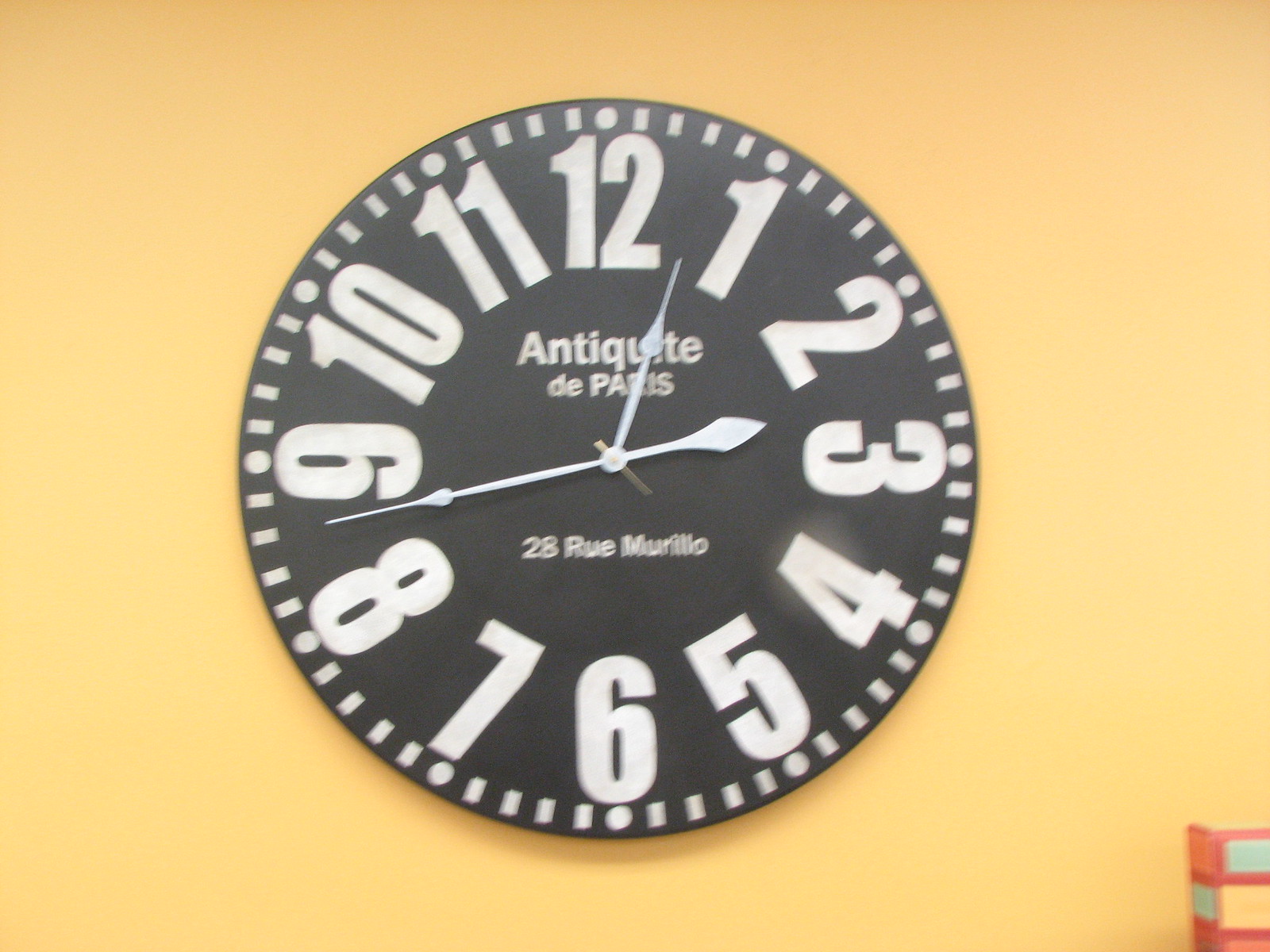This photograph features a striking black clock hanging on a vibrant mango-colored wall, which transitions from a darker tone at the top to a lighter yellow hue towards the bottom. The clock itself is circular, frameless, and has a minimalist design with bold, thick white numbers and white tick marks to denote the minutes. Prominently, the clock face reads "Antique de Paris" in the center, accompanied by the partial address "28 Rue" just below. The time is indicated by three white pointy hands: one each for hours and minutes, and a shorter one for seconds. To the right of the clock, there is a colorful, fluorescent orange cabinet or stacked drawer unit, featuring accents of green, yellow, and possibly a lighter shade of orange or another color like red, blue, and yellow. This bright and eclectic scene captures the stark contrast between the modern, monochromatic clock and the lively, multi-hued background and furniture.